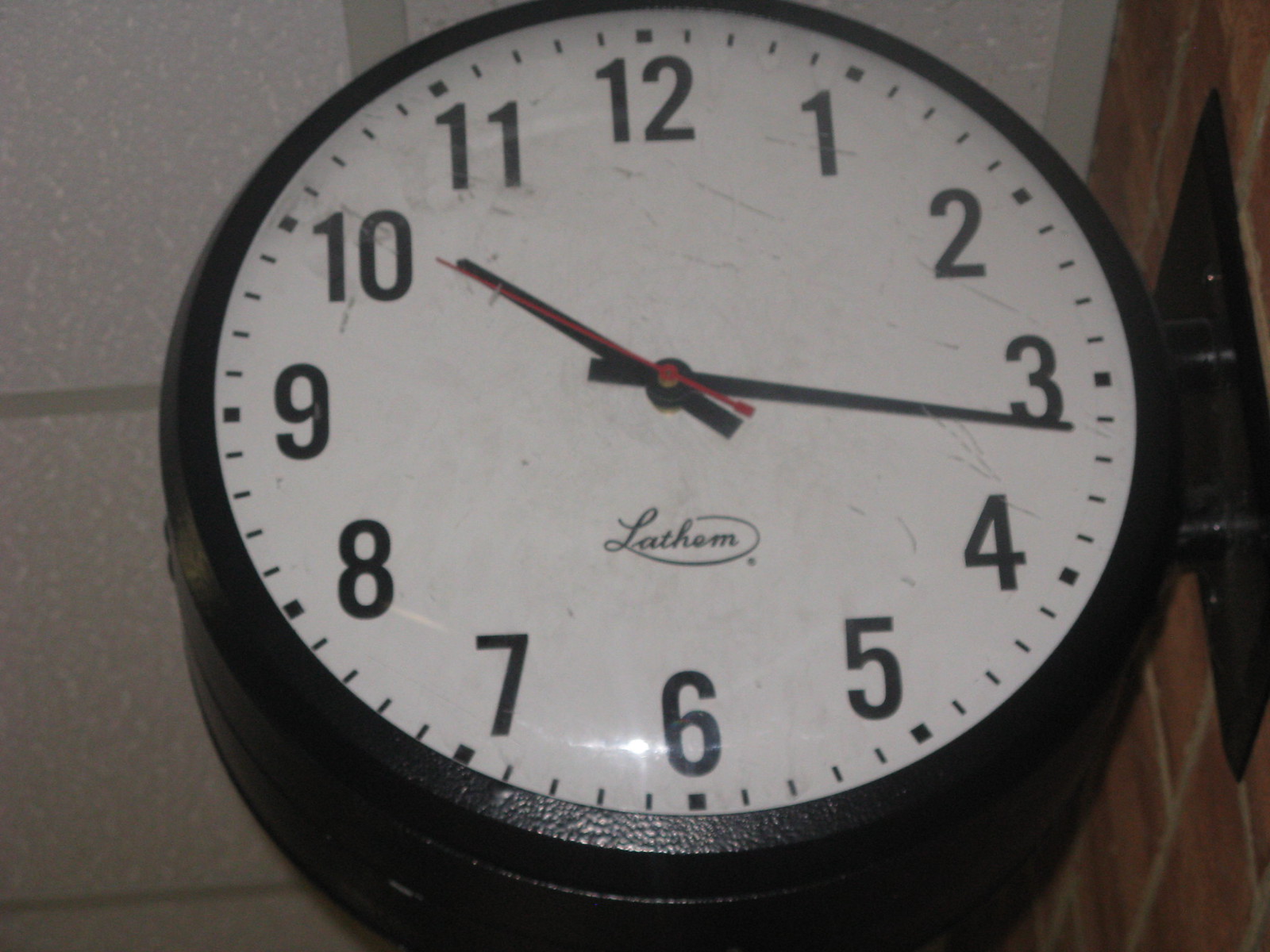The image depicts a close-up of a round clock mounted on a reddish-orange, brick-patterned wall. The clock has a white face with black numerals from 1 to 12, and black minute and hour hands, while the thin second hand is red. The clock is encased in a black, metal outer edge. It is attached to the wall with a black rectangular bracket and supported by two short cylinders, making it protrude slightly. The photograph also shows the white, tiled ceiling above with visible horizontal and vertical lines, and some cracks suggesting it's not a smooth surface. The time displayed on the clock is 10:16.